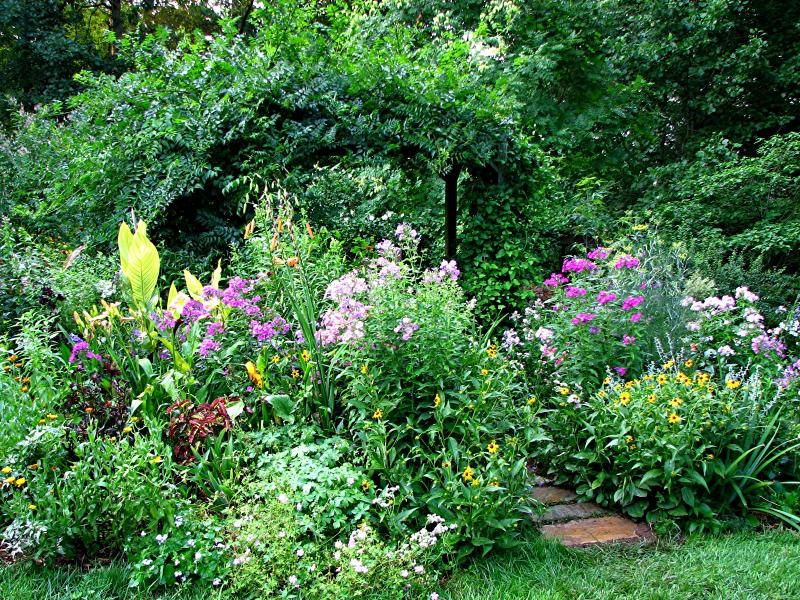The image captures an inviting outdoor flower garden with a well-kept grassy foreground and various vibrant flowers. The scene is dotted with black-eyed Susans, upright phlox, small white ground cover flowers, and variegated yellow-green leaf plants. Scattered throughout are yellow, pink, purple, and orange flowers, adding a colorful tapestry to the setting. The brick path meanders through the garden, composed of large bricks arranged in a row, leading the eye and foot through the lush greenery. Alongside the path and within the garden, taller shrubs and possibly variegated canna lilies rise, adding structure and height, while in the background, a manicured, lushly green area transitions into a small forested section. The path appears to continue under an arbor draped with wisteria, enhancing the garden’s enchanting atmosphere.